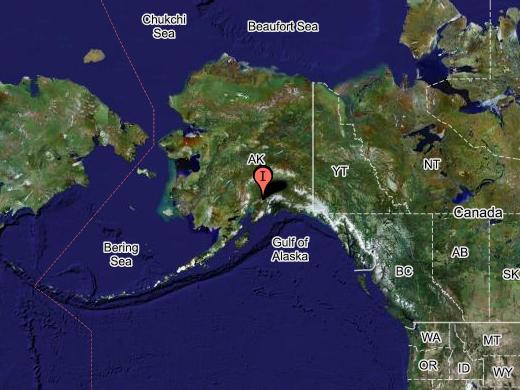A detailed AI-rendered digital map of Alaska viewed from space shows the state prominently in the center of the image, with parts of Canada and the United States in the lower right-hand quadrant. The map features the deep blue waters of the Gulf of Alaska, the Bering Sea, the Chukchi Sea, and the Beaufort Sea. The surrounding regions include the Yukon Territory, British Columbia (BC), Alberta (AB), Northwest Territories (NT), and potentially Nunavut (NU) in Canada. US states visible on the map include Washington, Montana, Oregon, Idaho, Wyoming, and small portions of Nevada and California. Notably, a red location pin marked with the letter "I" is dropped over an unnamed town in Alaska, suggesting something significant at that spot. A red border line separates Alaska from the nearby landmass of Russia, which is also partially visible. The map's terrain is shown in green with some white indicating elevations and ice caps, and areas are labeled with state and provincial abbreviations, such as "AK" for Alaska.